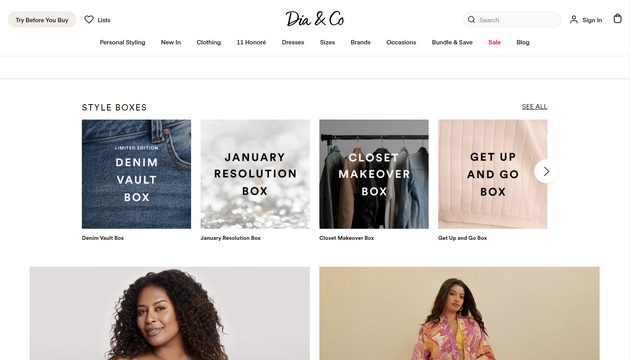**Screenshot of Dia & Co Website**

This screenshot captures the homepage of the Dia & Co website, a company stylized as Dia & Company (Dia is spelled D-I-A, and the 'and' is represented by an ampersand &). In the top left corner, there's a tagline "Try Before You Buy." Adjacent to that is a heart icon next to the word "Lists." Over on the right side, there is a search bar, a "Sign In" link, and a shopping bag icon.

The main navigation menu at the top includes options: Personal Styling, New In Clothing, 11 HONORE, Dresses, Sizes, Brands, Occasions, Bundle and Save, Sale, and Blog. Further product categories listed include Style Boxes, Limited Edition Denim Vault Box, January Resolution Box, Closet Makeover Box, and Get Up and Go Box.

The center of the page features two prominent photographs. The first is of a Black woman with long, wavy hair smiling directly at the camera. The second image features a young Latina woman with long, dark, wavy hair, dressed in a patterned blouse with yellow, white, and pink colors.

The image is horizontally oriented, being wider than it is tall, and contains no animals, buildings, plants, flowers, or trees.